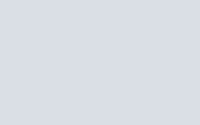This image depicts a small, gray square with a soft heather texture. Set against a white background, the square is uniform in color and shape, resembling a miniature rectangle. The simplicity of the gray square stands in contrast to the stark white environment, highlighting its soft hue and precise, clean edges. This visual can serve various purposes, such as a placeholder or a minimalist design element.